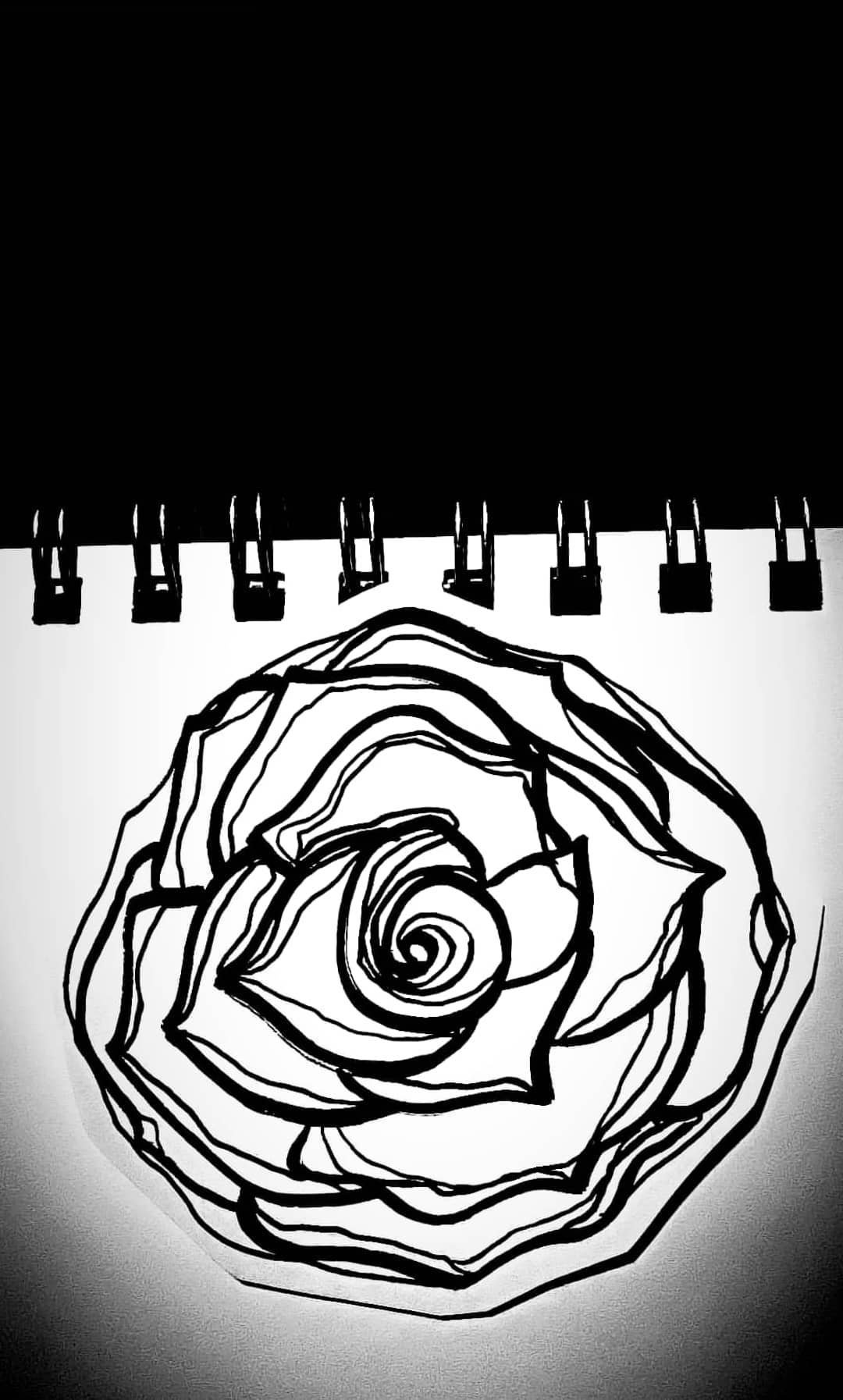The photograph showcases a black-and-white image of an artist's sketchbook set against a dark background. The sketchbook, lying in the lower half of the image, features the visible spirals binding the pages. Centered on the white paper is a detailed outlined drawing of a rose in full bloom. The rose is intricately rendered with black pen or marker, displaying multiple layers of petals that spiral outward from the center, some lines thick and some fine, creating a textured effect. The sketch lacks color and any accompanying text or print. Closer inspection reveals that the rose drawing appears to be a cutout, placed atop the sketchbook page, as evidenced by visible edges and slight shadowing on the lower right-hand side. The image is monochromatic and well-focused, with slight shadowing in the lower corners, possibly suggesting a directional light source emphasizing the details of the rose and the sketchbook layout.